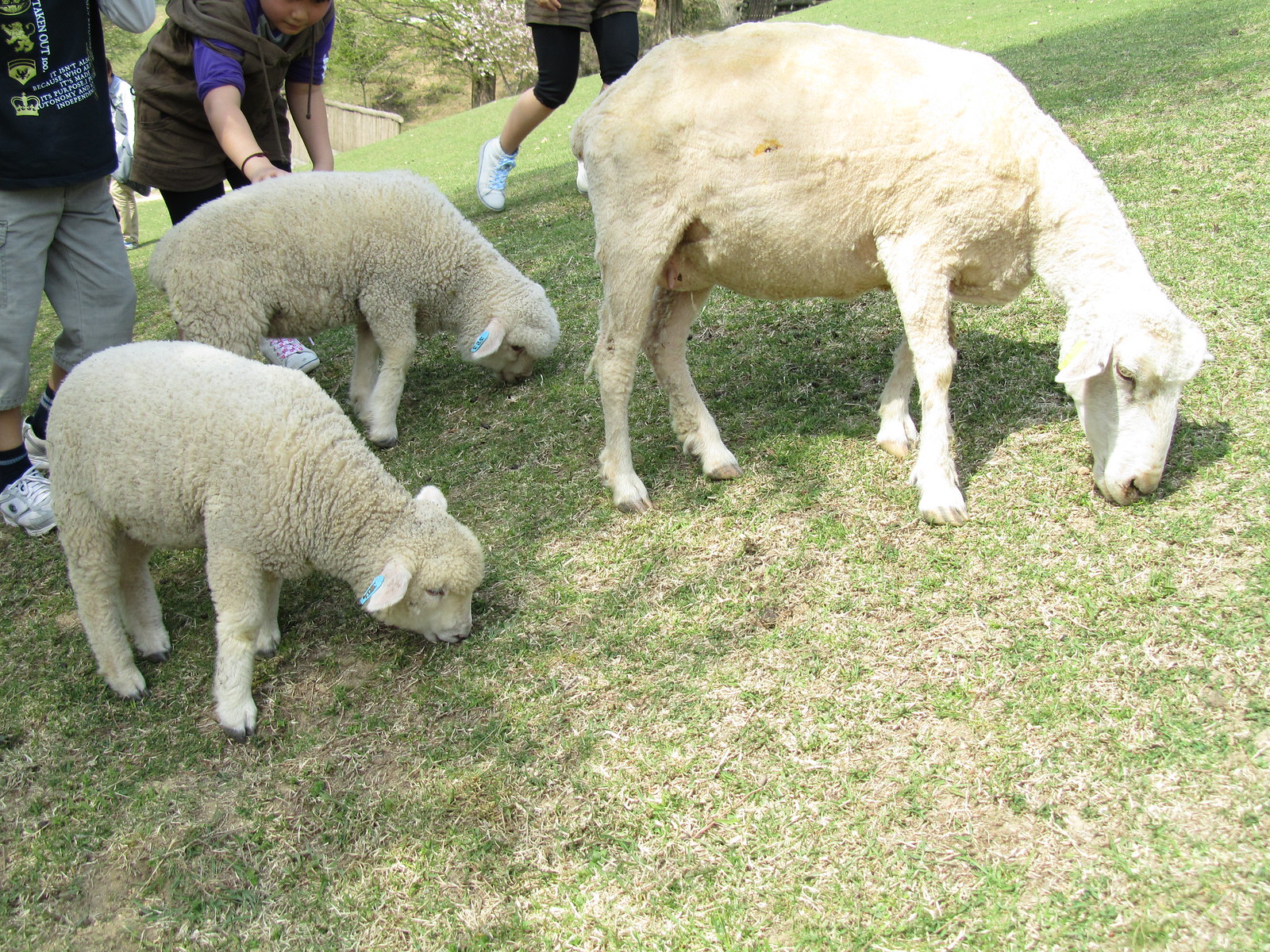In this vibrant daytime photograph, three white sheep are depicted grazing on a gently sloping grassy hill, which features patches of green interspersed with dry, brown areas. The sheep are organized such that the adult, identified as the mama sheep, stands in the foreground on the right, with her two fluffy, wool-covered lambs lined up behind her. The mama sheep has been freshly sheared, presenting a stark contrast to the full, dense wool coats of the lambs. All three are engrossed in feeding, their heads bent low to the ground.

Behind the sheep, a few people are visible, possibly part of a petting zoo setting or a casual farm visit. One person, dressed in a brown sweater layered over a blue shirt, is bent over petting one of the lambs. Another is in the background wearing a black shirt with tan capris and white shoes. The third individual appears to be someone in shorts and leggings. The hill they are on is part of a larger, neighborhood-like area, as suggested by the partial view of a house or a fence, and the presence of trees adorned with white blossoms. Sunlight casts soft shadows on the scene, enhancing the warm and cheerful atmosphere of this delightful outdoor moment.